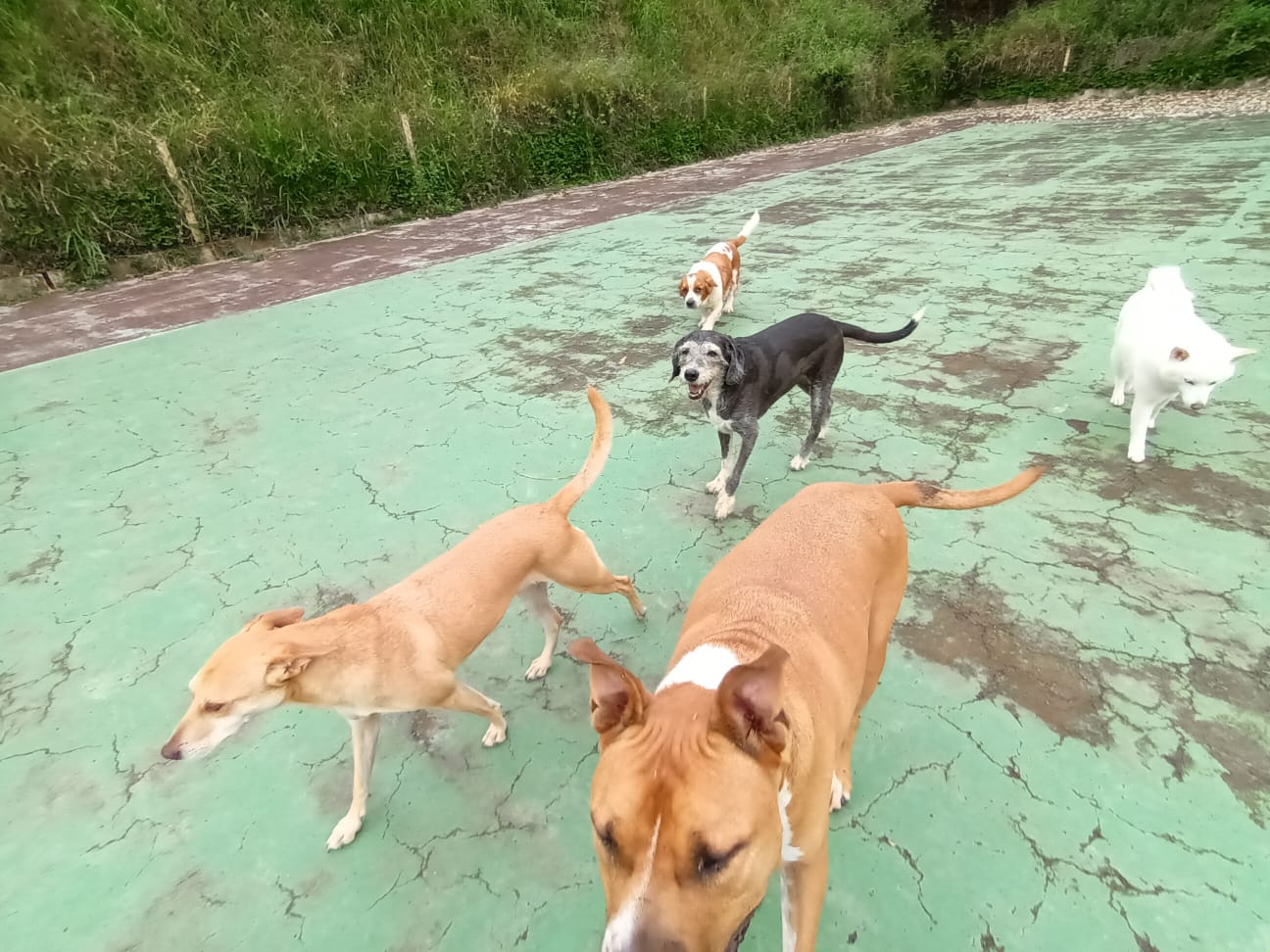This photograph captures a group of five dogs walking on a cracked and weathered green concrete surface in what seems to be a parking lot. The concrete is visibly worn and surrounded by very tall, thick grasses, about three feet high, nearly overtaking some fence posts in the background. 

Leading the pack is a dog that looks like a pit mix, his nose slightly cropped out of the frame, standing or leaning toward the person taking the picture. Following him is a beige dog, a mostly black dog with a white and gray speckled face, white feet, and a white chest. This black dog also sports a white-tipped tail. 

Next, there is a white dog that resembles a Husky positioned on the far right. Among the group is also a Jack Russell-looking dog positioned on the left. The pack includes another tan dog with white markings on its neck and part of its nose and pointy ears. A final paler tan dog with white feet and a white muzzle completes the lineup. All the dogs are off their leashes, yet they appear to be following the same unseen person in an orderly fashion, heading in the same direction.